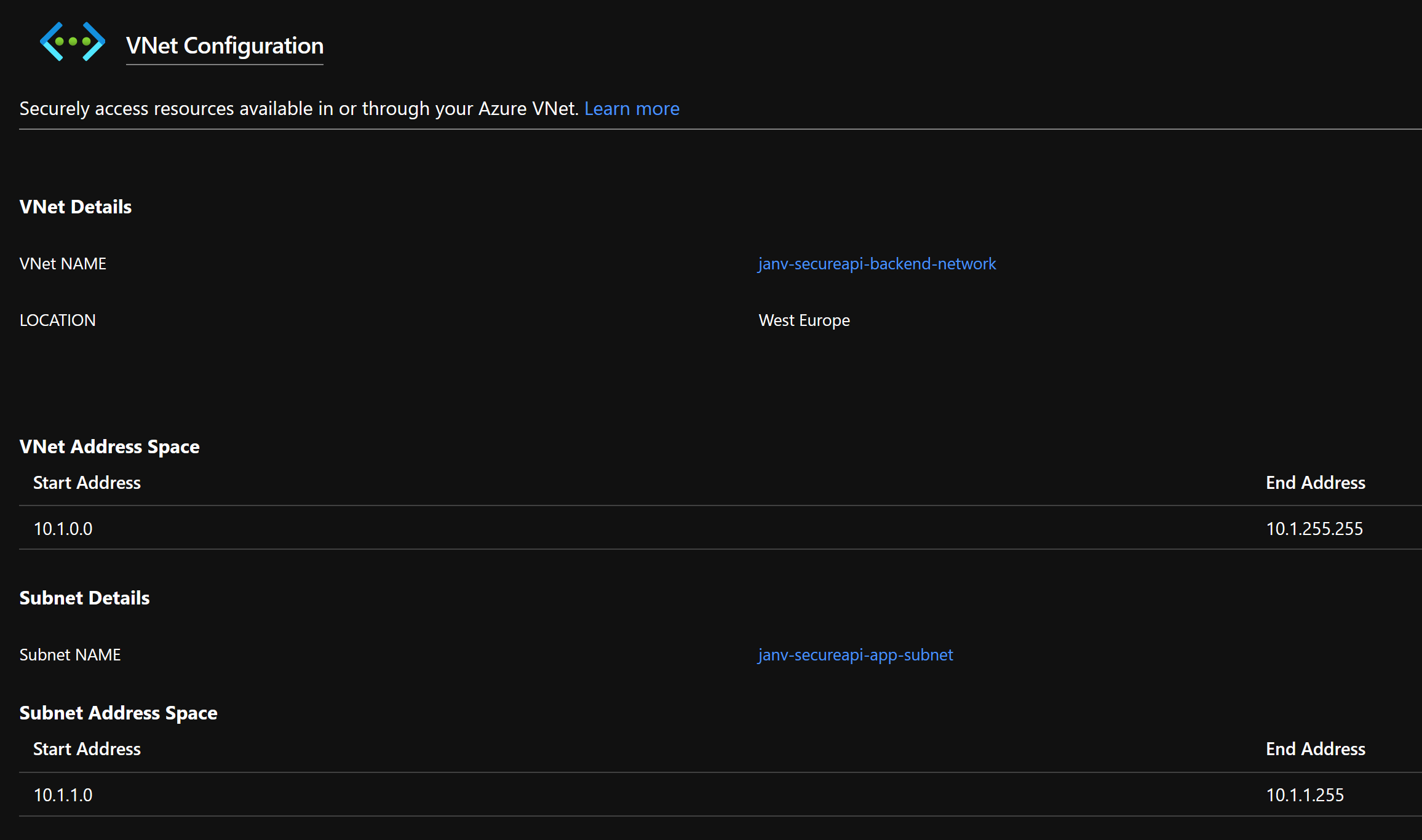This image provides a detailed configuration overview of an Azure VNet. The backdrop is black, enhancing the prominence of the visual elements. Centrally positioned, there's a symbol comprising blue arrows pointing left and right with three green dots interspersed between them, underscoring network connectivity.

Below the symbol, a message reads: "Securely access resources available in or through your Azure VNet. Learn more." This is followed by sections detailing the VNet's specifications.

1. **VNet Details:**
   - **VNet Name:** Jan V Secure API Backend Network
   - **Location:** West Europe
2. **VNet Address Space:**
   - **Start Address:** 10.1.0.0
   - **End Address:** 10.1.255.255

3. **Subnet Details:**
   - **Subnet Name:** janv.secureapi.app.subnet
   - **Subnet Address Space:**
     - **Start Address:** 10.1.1.0
     - **End Address:** 10.1.1.255

At the top, a "Learn more" button is available for additional guidance on configuring and leveraging Azure VNet. This comprehensive depiction simplifies understanding the VNet setup and assists users in tailoring the network to their specific requirements.